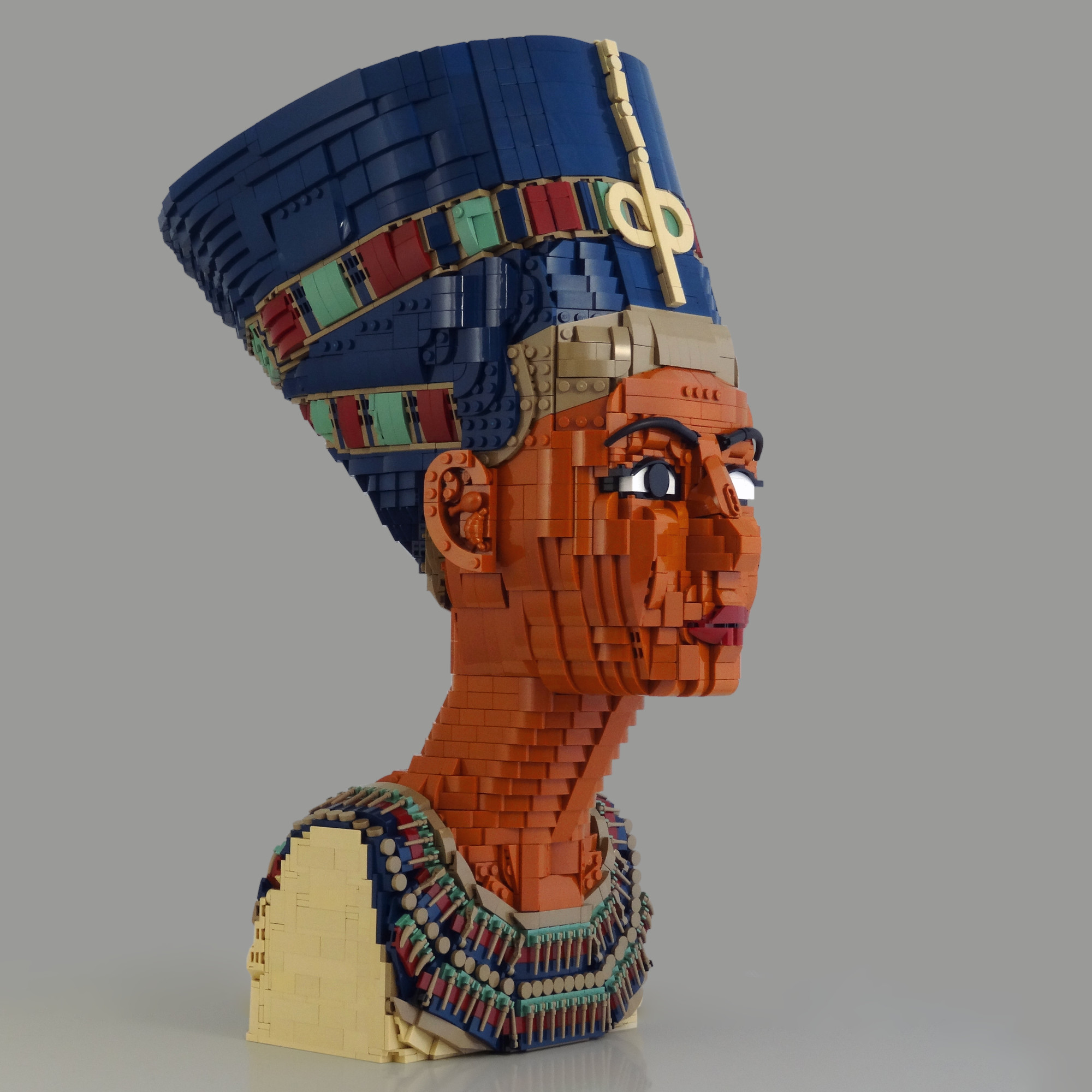The image depicts a highly detailed LEGO bust of Nefertiti against a solid black or gray background. The sculpture, made entirely of LEGO bricks, showcases Nefertiti with a distinct stair-step texture characteristic of LEGO creations. She has a darker skin tone, black eyes, and red lips that stand out. Nefertiti is adorned with an elaborate headdress that is predominantly blue and intricately accented with red, dark blue, teal, and yellow decorations. Her head wrap, which complements the necklace, features a similar color palette. The necklace drapes over her shoulders with green, red, and blue beads, matching the hues in her headdress. The bust, capturing Nefertiti's long neck and detailed facial features, conveys a regal and historical essence through its meticulous LEGO artistry.